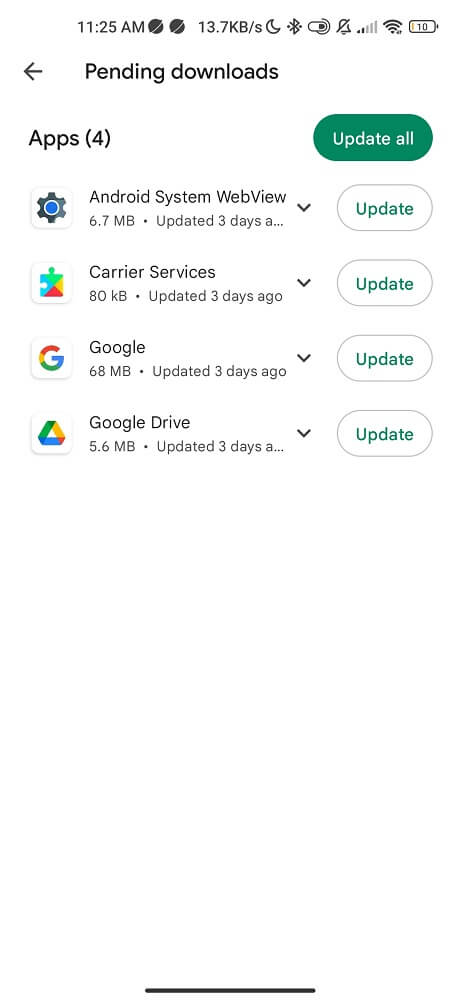The image captures a mobile screenshot showcasing a list of applications pending updates on a device. At the top of the screen, set against a white background, is the heading "Pending downloads" in black text, accompanied by a left-pointing arrow for navigation. Below this heading, there is a section labeled "Apps" with the number (4) in parentheses, indicating the quantity of apps needing updates. To the right side of this label is a green button with white text that reads "Update all."

The main portion of the screenshot displays four applications listed one after another. Each app is accompanied by its icon on the left side, followed by the app's name: "Android System WebView," "Carrier Services," "Google," and "Google Drive." Below each app name, additional information is provided, such as file size and the time frame since the last update. For "Android System WebView," it displays "6.7 MB, updated three days a..." which is cut off. Similarly, "Google Drive" reads "5.6 MB, updated three days a..." before truncating. Both of these entries feature a small black downward caret and a white button with a gray outline inscribed with "Update" in green. The "Carrier Services" app shows "80 KB, updated three days ago," and "Google" denotes "68 MB, updated three days ago," with both entries also featuring the same caret and update button arrangement.

The bottom portion of the image shows significant white space, with a thin horizontal black line near the very edge, typical of mobile device design elements. At the top of the screenshot, the device's status bar displays various icons: the time reading 11:25 AM, two black circles with white vertical dashed lines, a data rate indicator showing "13.7 KB/s," a crescent moon symbol (likely for do not disturb mode), Bluetooth, vibration/silent mode (illustrated by a bell with a slash), Wi-Fi signal strength, and a battery icon showing "10" with a minimal yellow strip, indicating only 10% battery life remaining.